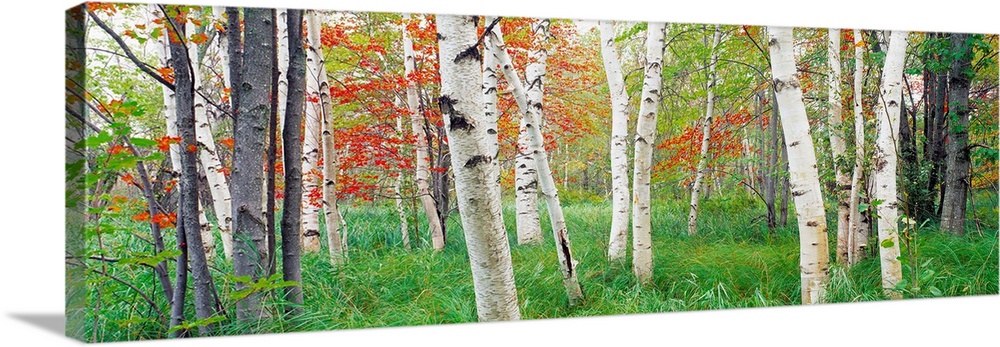This is a vivid 3D landscape photograph reproduced on a long, horizontally-stretched rectangular canvas, perfect for wall hanging. The scene captures the essence of a transitional season, likely fall, in a dense woodland area. Dominating the foreground are tall, slender birch trees characterized by their distinctive white bark adorned with brown or black spots. Interspersed among the birches are various dark brown and dark gray tree trunks. The vibrant ground is covered in overgrown, tall green grass, adding a lush texture to the scene. The background reveals a colorful tapestry of foliage with leaves in radiant shades of green, red, and orange, indicative of the changing seasons. The bright, vivid colors saturate the photograph, enhanced by the apparent sunlight filtering through the canopy, giving the entire piece a lively and dynamic depth.